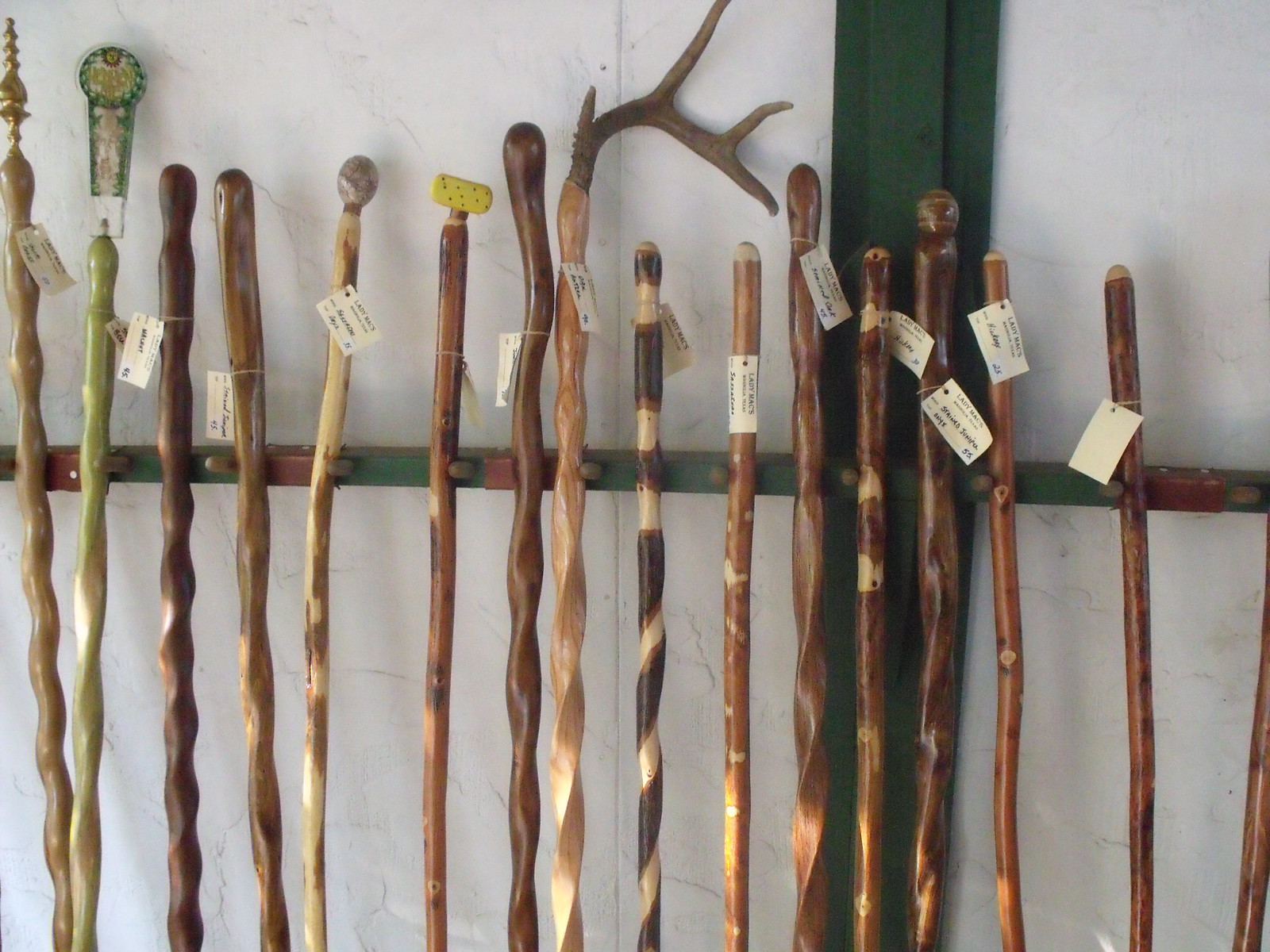In this indoor image, we see an array of hand-carved wooden walking sticks meticulously displayed against a white wall with green trim and an upraised horizontal green shelf. Each unique walking stick bears a small tag, presumably indicating their prices. In total, there are 16 walking sticks, varying in design and color. Some sticks are straight, while others have intricate twists, some featuring two types of wood intertwined. Notably, one stick on the left is painted green, another in the middle has a spiky handle which wouldn’t be practical for holding, and another in the middle features a curved antler handle. Each stick, separated by small knobs to prevent touching, showcases a spectrum of craftsmanship from light golden hues to dark polished finishes.